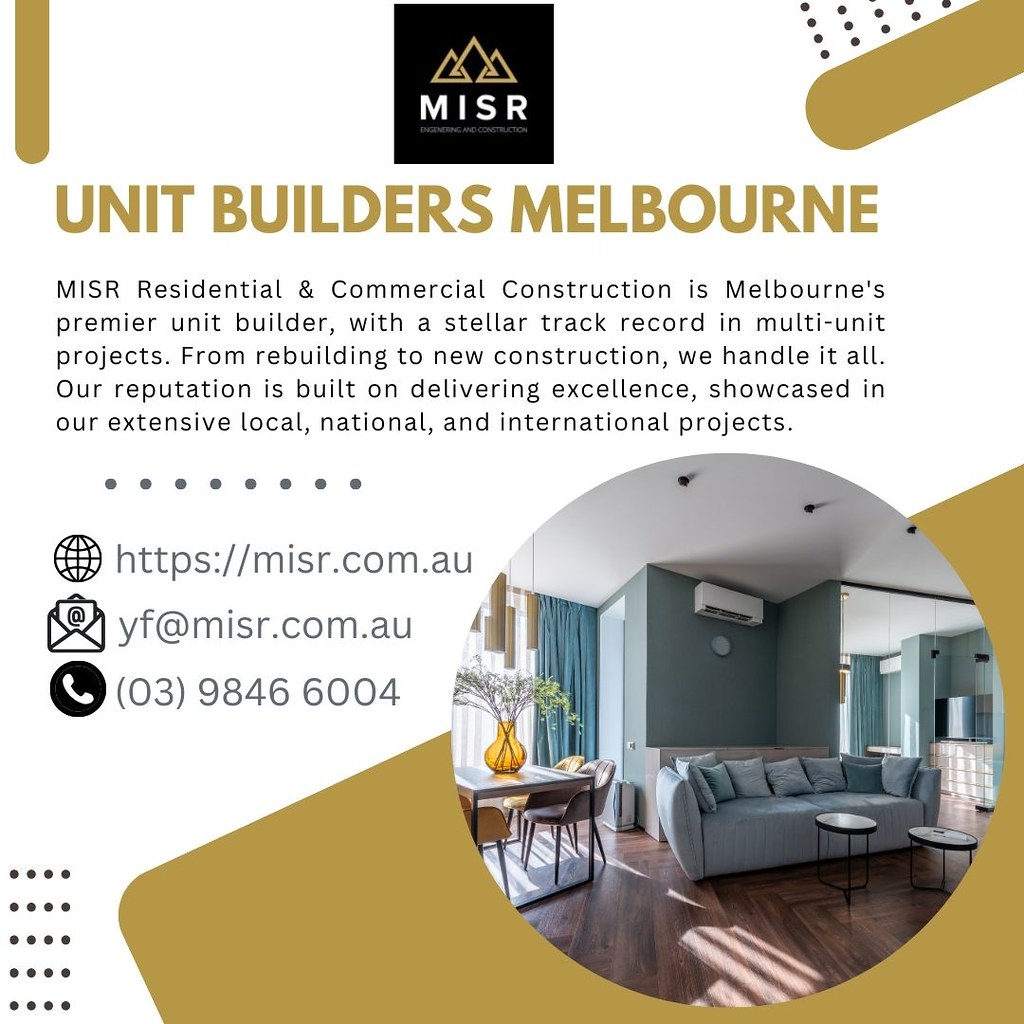This image, likely an advertisement for MISR Unit Builders in Melbourne, features a meticulously designed layout with a white square background. The top-middle prominently displays the MISR logo, a black square with three gold triangle mountains above it, and "MISR" in white capital letters. Directly below the logo, in gold letters, the text reads "Unit Builders Melbourne." 

Beneath this, a detailed description in black text outlines MISR's expertise in residential and commercial construction, emphasizing their reputation in handling a wide range of projects, from renovations to new constructions, both locally and internationally. 

Adjacent to this text, contact information is provided, including their website (https://www.misr.com.au), email (YF@misr.com.au), and phone number (03 9846 6004).

On the right side of the advertisement, there is a circular photograph showcasing a beautifully decorated living room, featuring a gray sofa, gray walls, turquoise curtains, and a couple of small end tables. This interior image is accented by a gold, slanted box-like design, adding a touch of elegance and cohesion to the ad's overall aesthetic.